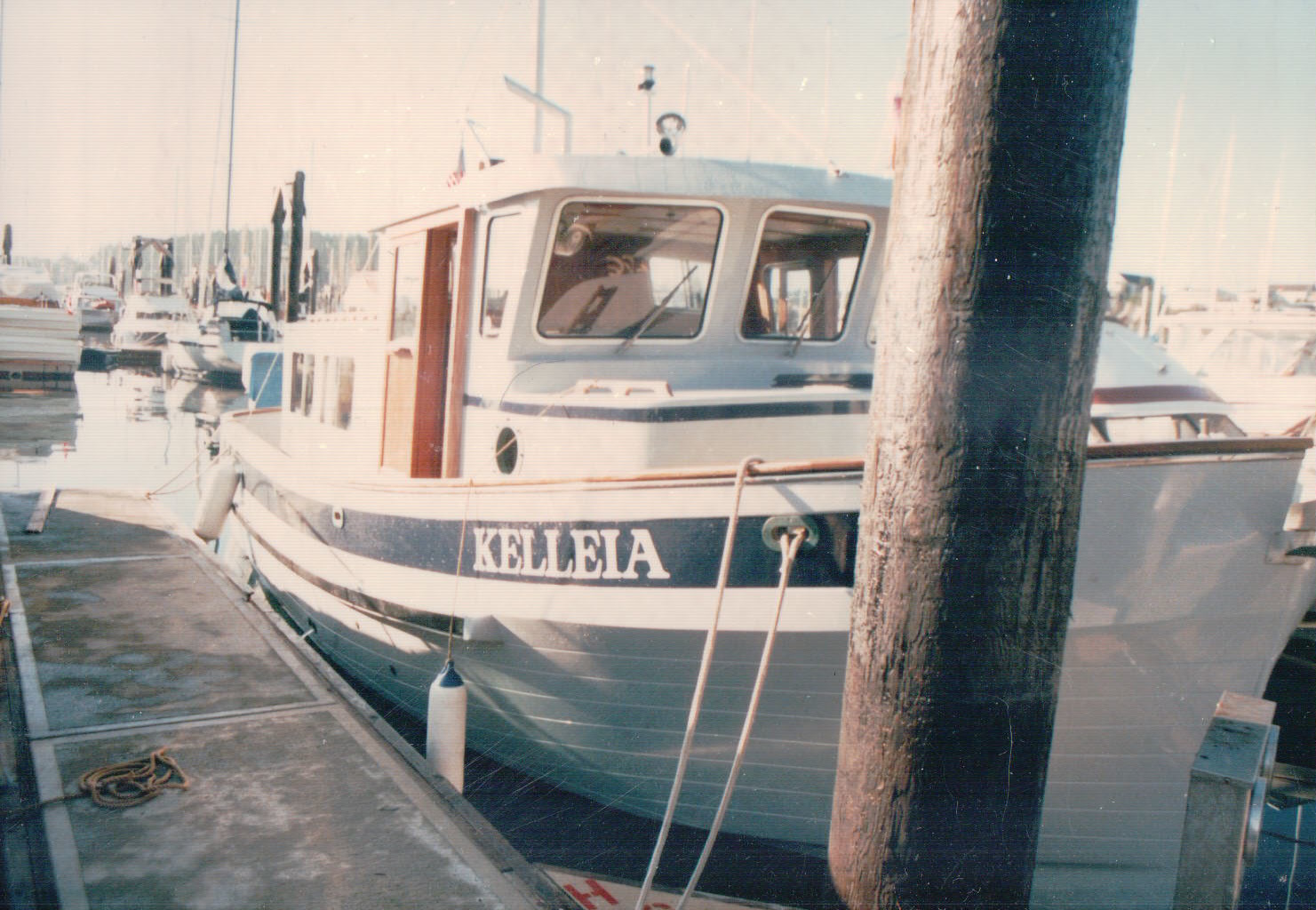This photograph, likely taken in the 1970s or 80s given its brownish-yellow tone and grainy quality, captures a quaint docking site for various boats, including yachts and riverboats. The focal point is a small cruise boat named "KELLEIA," with its name emblazoned in white letters on a blue stripe along its side. Predominantly navy and white, with a distinctive red door, the boat features an upper deck where the captain navigates and passengers can enjoy the view. A wooden pole connected to the concrete pier prominently occupies the foreground, partially obstructing the view but adding to the vintage ambiance. Surrounding the "KELLEIA" are several smaller sailboats, all moored on the water, enhancing the tranquil, timeless feel of the scene.